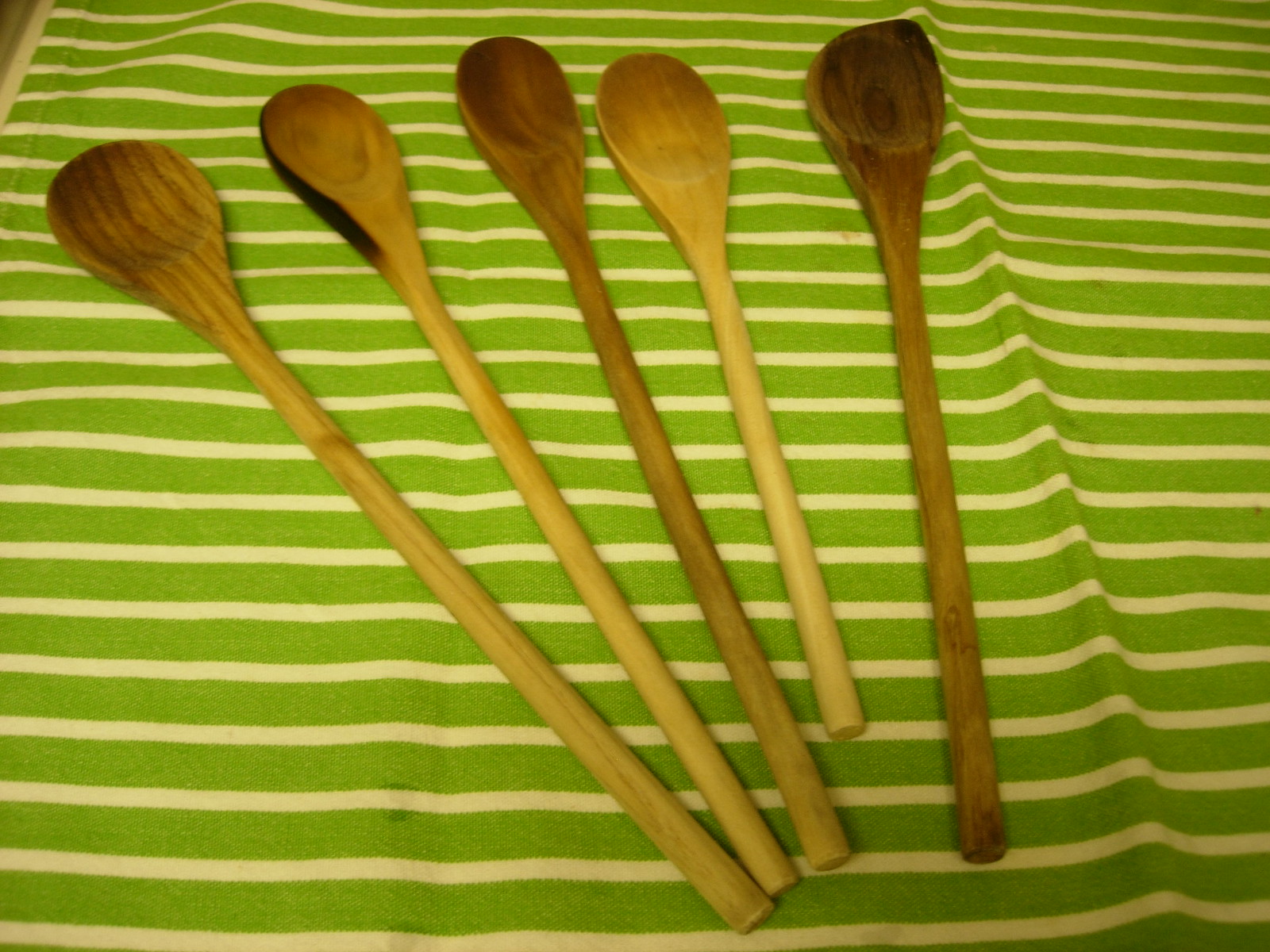In this close-up image, five wooden kitchen spoons are artfully arranged on a green and white striped kitchen towel, which is neatly folded with a visible crease down the middle. The spoons, varying in size and wood grain, are angled towards the left side of the picture, with their spoon portions positioned at the top and handles pointing towards the bottom right center. 

The first spoon, to the far left, is the largest with a wider spoon section and features a darker wood grain at the top, transitioning to a lighter handle. The second spoon has a slender spoon end with a distinctive brown burn mark along its side, and also has a lighter handle. The third spoon displays a uniform, darker wood grain and is considered a standard wooden spoon. The fourth is shorter and made of lighter wood, reflecting a simpler design. Finally, the spoon on the far right is notable for its unique tip that points to the right, maintaining a rounded spoon part; it is the darkest in overall wood grain, extending from the spoon part to the handle. The vibrant green towel with white stripes provides a contrasting backdrop that highlights the varied shades of the wooden spoons.